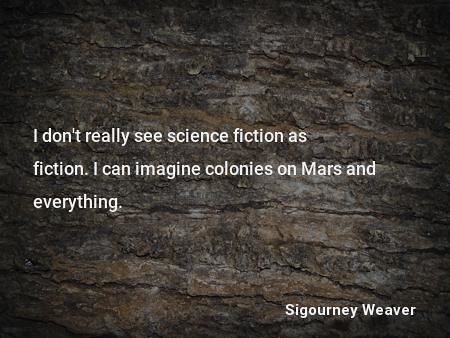The image features a close-up photograph of grayish-brown bark with distinct horizontal ridges, suggesting either the bark of a tree or a piece of wood. The background, which is textured and darkens towards the edges, evokes the natural, rugged appearance of stone. Printed in the center of the image in white text is a quote from the actress Sigourney Weaver: "I don't really see science fiction as fiction. I can imagine colonies on Mars and everything." Sigourney Weaver's name is also printed in the same white text at the bottom right corner of the image. The overall composition of the photograph is a horizontal rectangle, slightly wider than it is tall. This striking blend of natural texture and thoughtful quotation emphasizes both the organic and imaginative aspects of Weaver's perspective on science fiction.